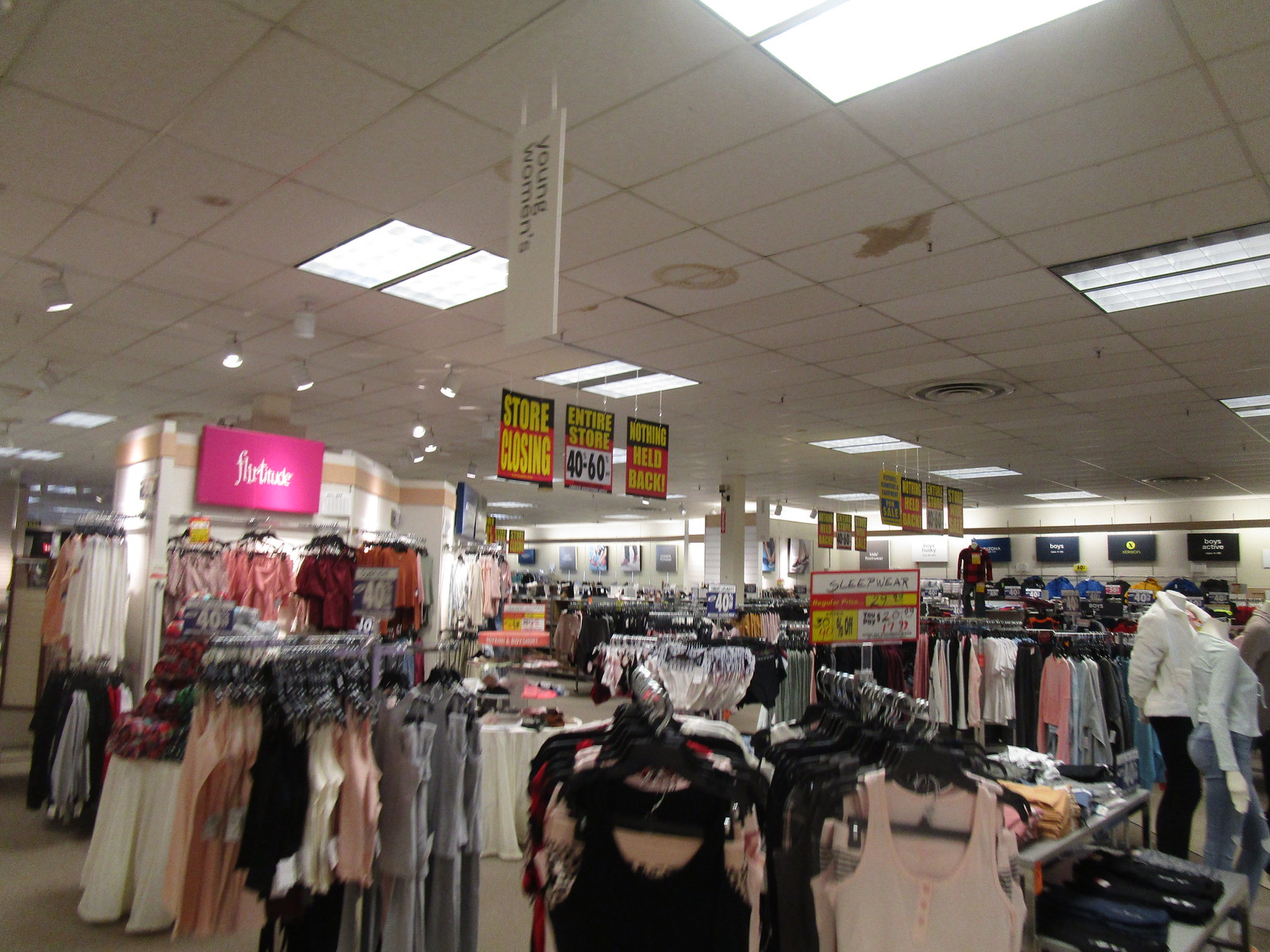The image depicts a large department store in the process of closing down. The ceiling, adorned with white tiles, shows multiple stains and features an air vent. Natural light streams in through several large windows. Numerous signs hang from the ceiling; most of them are black and orange with yellow writing, announcing store closing sales. Prominent among them is a sign indicating discounts of 40 to 60 percent off. The store is filled with various sales signs.

In the foreground, several large racks of women's clothing are displayed, with a notable pink sign displaying the word "Future". There are at least four racks of tops visible. In the background, the dressing rooms can be seen, suggesting this area was once bustling with shoppers trying on clothes. The overall atmosphere captures the final days of the store, marked by significant discounts and an impending closure.